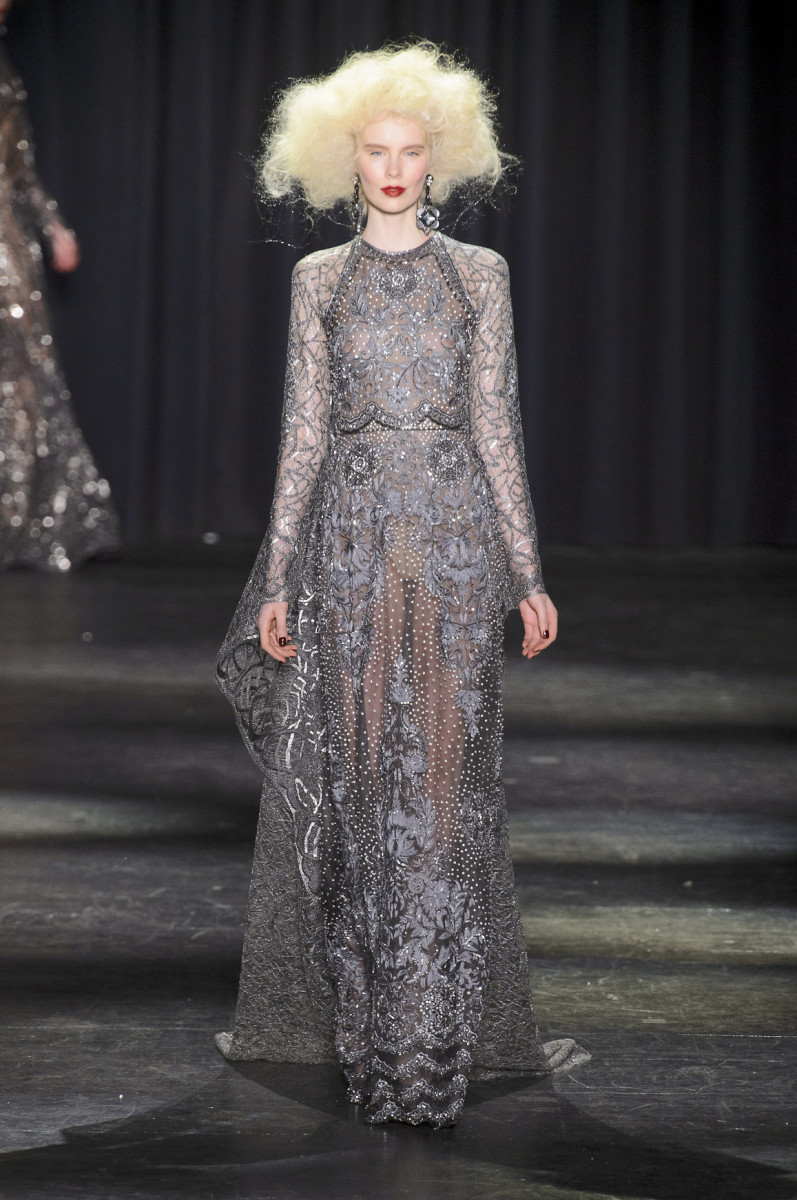A tall, pale model with poofy, messy, light blonde hair, possibly a wig, is walking down a dark gray runway during a fashion show. Her hair is reminiscent of a cotton ball, deliberately unkempt. She is wearing a long, semi-transparent, ornate gown adorned with argyle-esque embroidery in shades of gray, white, and black. The dress is highly detailed, revealing the faint outlines of her legs and arms through the fabric, while the sleeves are even more transparent. She has striking red lipstick and black fingernail polish, adding contrast to her look. Black flower-like earrings dangle from her ears, enhancing her dramatic appearance. The runway is well-used and lit by spotlights, with black curtains in the background. Another model in a similar attire is visible in the distance, about to follow her. The model in focus continues to command attention, looking directly towards the camera, letting the crowd, which remains unseen, take in the spectacle.